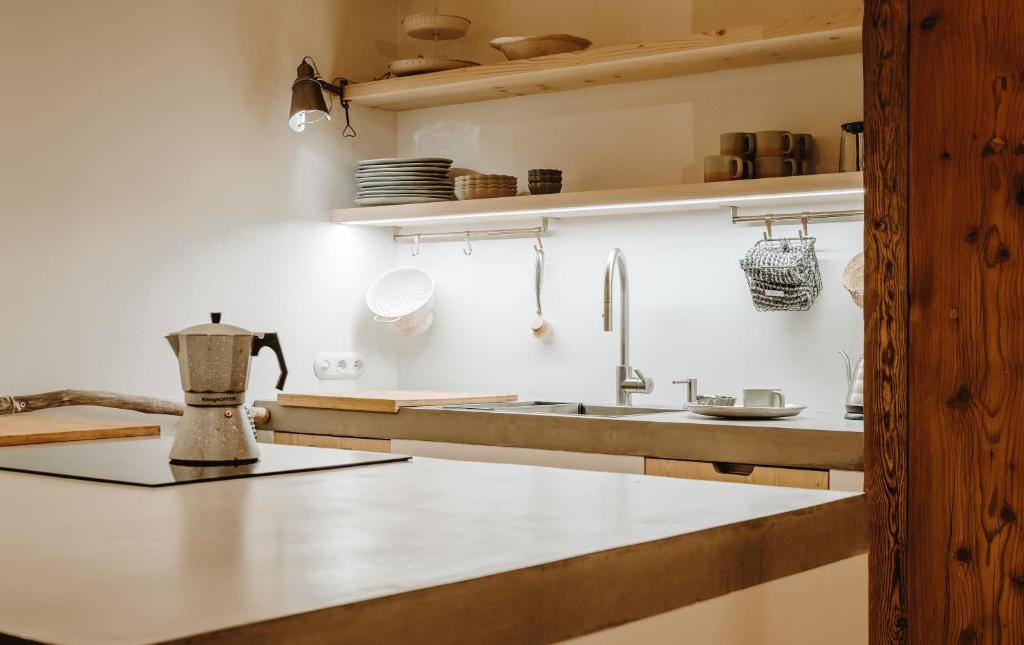The image depicts a simple and brightly lit kitchen with white walls and light brown cabinets and shelving. In the foreground, there is a large island with tan countertops, featuring a silver coffee pot with a black handle and top, as well as a cutting board. Behind the island, to the right, there is a metal faucet above the sink, next to which sits a white plate with a white cup, possibly holding a piece of pie. Above the sink, two shelves contain a neat stack of about 10 white plates, several small bowls, and some coffee cups. Additionally, a clamped light fixture on one of the shelves illuminates the area below. To the left of the sink, there are some items hanging on the off-white wall. The overall setting suggests a kitchen that could be located in a foreign country based on its distinctive look.